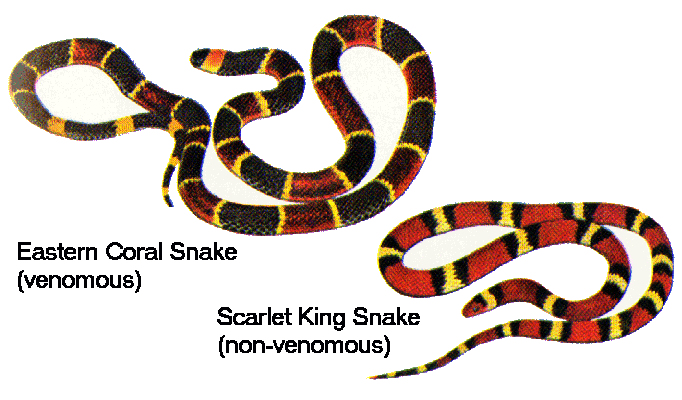The illustration features two snakes on a white background. In the top left, the Eastern Coral Snake, labeled in black text with "(Venomous)" beneath its name, is depicted with a distinctive pattern of thick black bands separated by thin yellow stripes. This larger snake coils in a complex path: curling left, then down and to the right, up, down, left, then up and left again, finally coiling back to where its head rests. Its alternating yellow and red coloring adds to its vivid appearance. 

Positioned in the bottom right is the smaller Scarlet King Snake, labeled with "(Nonvenomous)" next to its name in black text. This snake features a pattern where its primary color is red, interrupted by black bands separated by small yellow rectangles. It curls with its tail starting at the bottom center of the frame, moving up and to the right, then up, left, down, right, down, and finally left where its head, marked by a blue eyeball, is located. The Scarlet King Snake is notably smaller in both diameter and length compared to the Eastern Coral Snake.